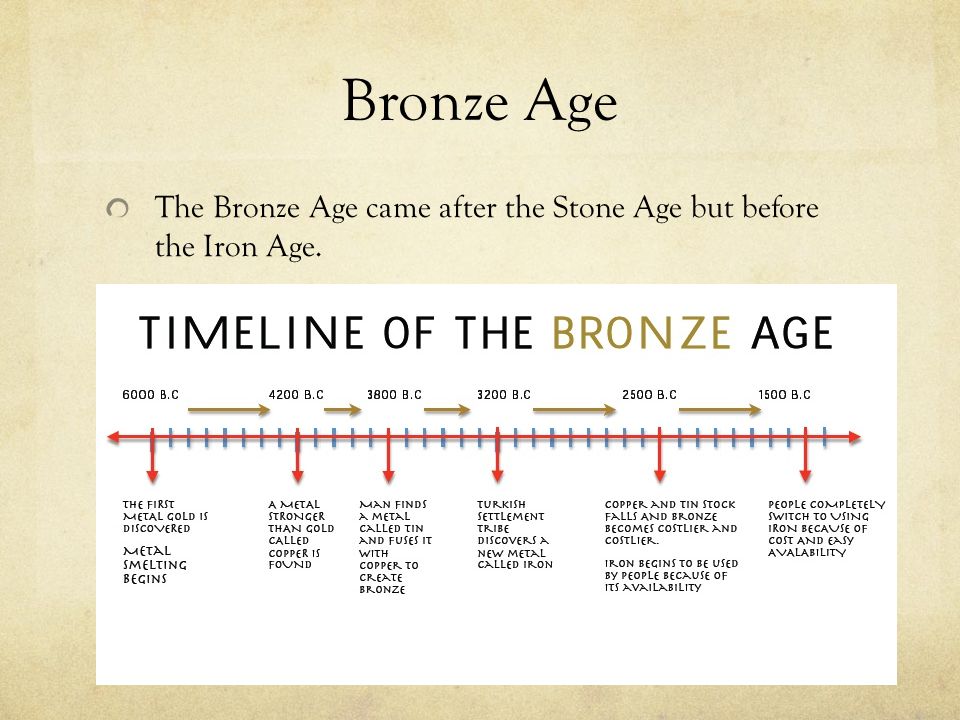This image is a detailed educational poster with a cream, parchment-colored background, featuring information about the Bronze Age. At the top, in bold black writing, the title reads "Bronze Age". Below that, in a smaller typeface, it states, "The Bronze Age came after the Stone Age but before the Iron Age."

Dominating the center downwards is an inset image with a white background displaying a timeline titled "Timeline of the Bronze Age." The timeline provides key milestones: 

- 6000 BC: The first metal, gold, is discovered and metal smelting begins.
- 4200 BC: Copper, a metal stronger than gold, is found.
- 3800 BC: Tin is discovered and fused with copper to create bronze.
- 3200 BC: A Turkish settlement tribe discovers iron.
- 2500 BC: Copper and tin stocks fall, making bronze increasingly costly, and iron begins to be used due to its availability.
- 1500 BC: People completely switch to using iron because of its lower cost and easy availability.